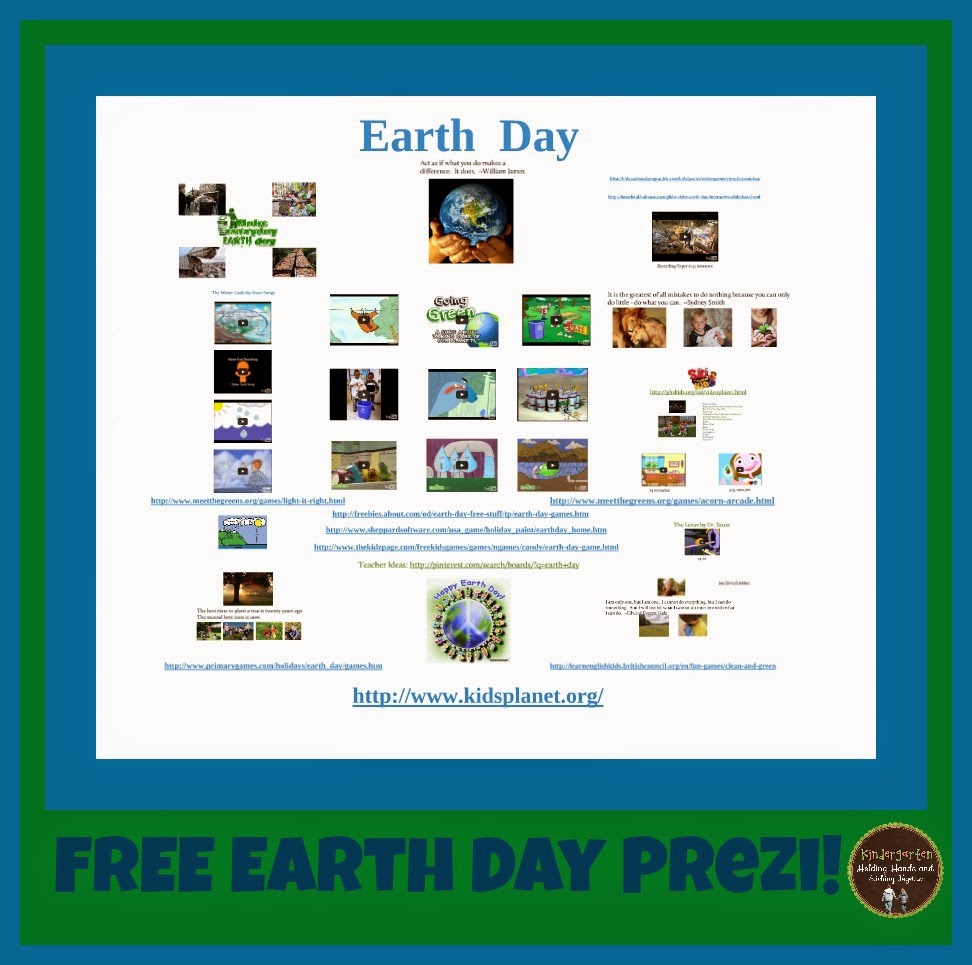"An intricately designed Earth Day promotional graphic featuring a central blue square with a green border. At its heart, the image showcases a globe being held delicately in someone's hands, symbolizing care for our planet. Surrounding the main visual, there are a series of smaller pictures and videos, providing informative content about Earth Day. These include depictions of people forming a circle around another globe, emphasizing community and global unity. The graphic joyfully proclaims 'Happy Earth Day,' and directs viewers to the website http://www.kidsplanet.org for more resources. Highlighted by a red circle, the promotion also advertises a free Earth Day present with detailed explanations. This vibrant and information-rich design aims to inspire and educate viewers about the importance of Earth Day celebrations."